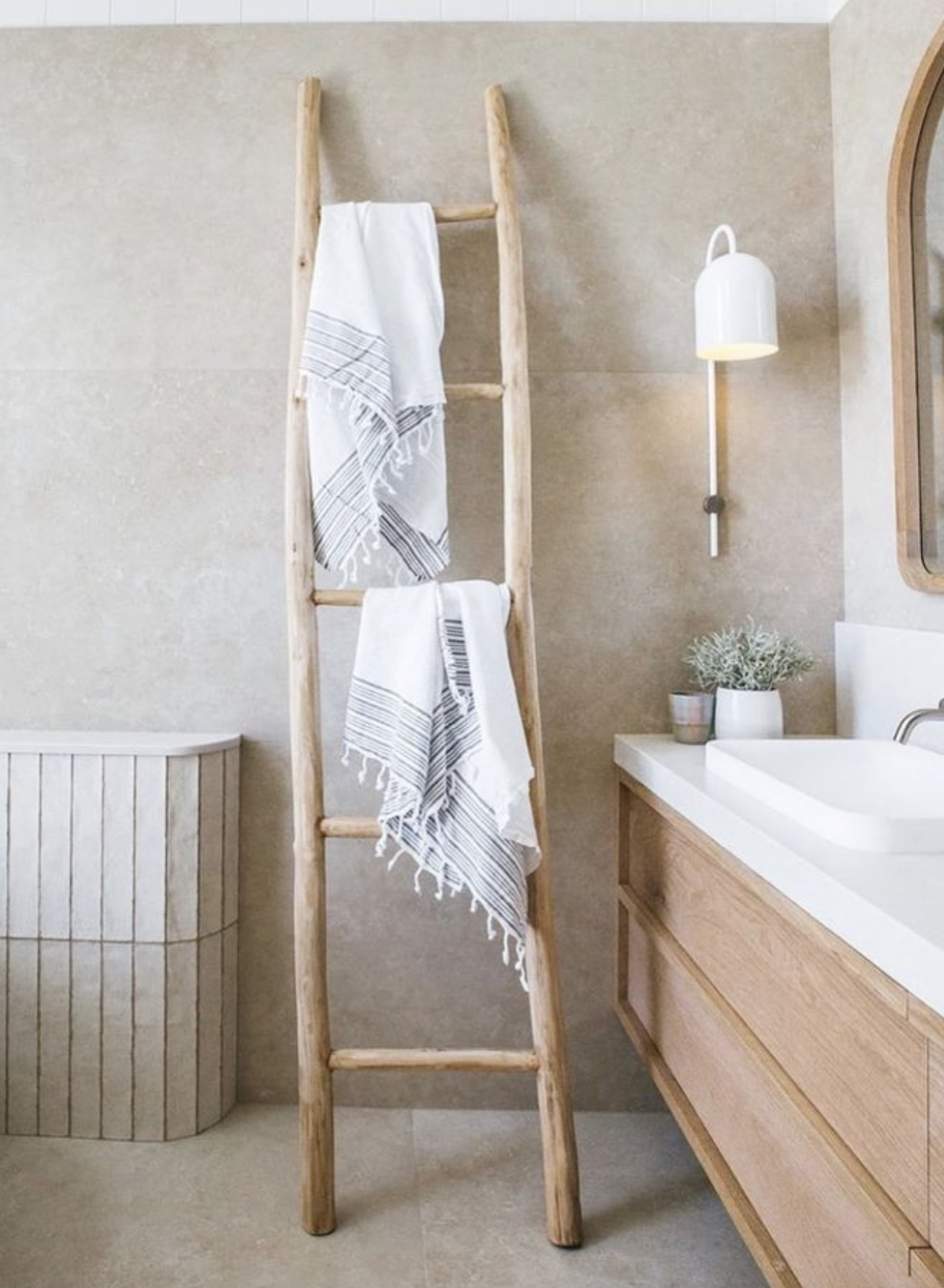The photograph captures a high-end bathroom featuring a decorative ladder that appears to have been meticulously crafted from rough-hewn tree branches and polished to a light brown hue. This ladder, leaning against a flat tan-colored wall and matching tan floor, functions as an elegant towel rack. Two white towels with black and gray striped ends are draped over different rungs, emphasizing its decorative use. To the right of the ladder, a white countertop supports a small white pot containing a vibrant green plant, alongside a chrome faucet and sink. Beneath the counter are light brown wooden cabinets. To the left of the ladder stands a light brown hamper, contributing to the room's cohesive earthy tones. Additionally, a wall-mounted light fixture above the countertop casts a warm glow, enhancing the sophisticated ambiance of the bathroom.